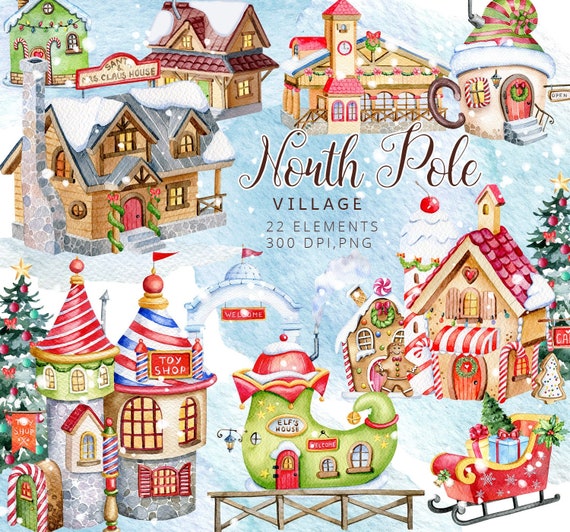This vibrant and cheerful Christmas poster, titled "North Pole Village," features a lively array of festive elements set against a blue background with white snow. The central text, written in brown letters outlined in gold, reads "North Pole Village," followed by "22 Elements" and "300 DPI, PNG." Surrounding this central text are numerous charming holiday scenes and structures. 

In the upper left corner, there is a quaint greenhouse adorned with candy canes by the door. Below it, you'll find the two-story house of Saint Santa and Mrs. Claus. To the bottom of the poster is the whimsical Elf's House, shaped like a shoe, adjacent to a beautifully decorated Christmas tree. Nearby, there’s a vibrant Toy Shop, distinguished by its cone-shaped roofs topped with round ornaments. To the right, a gingerbread house sits festively, complemented by another Christmas tree behind it. Additionally, there is a small sleigh filled with presents, adding to the holiday spirit. The entire image exudes a joyful and colorful atmosphere, making it a perfect depiction of a bustling, picturesque North Pole village.